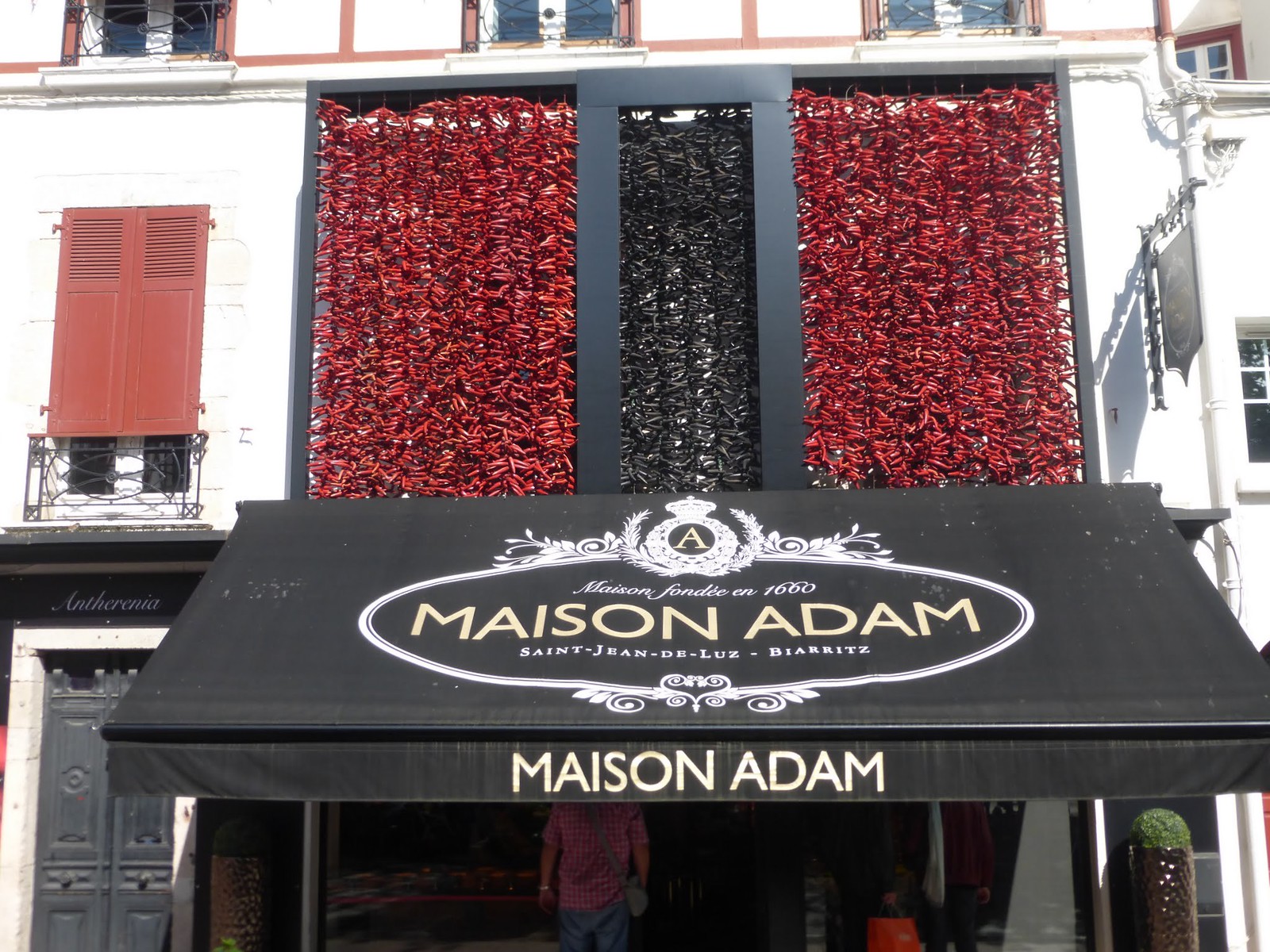In this image, we see the facade of a mostly white building adorned with a standout black awning. The awning prominently displays the text "Maison Adam" in yellow and "St. Jean de Luz" in white. Below these, "Biarritz" is also inscribed in white. The entrance, framed in what looks like a black or gray door, appears ready to welcome visitors, with a person visible, possibly walking out. 

The building is further accentuated by numerous red shutters that pop against the white backdrop. Sunlight brightens the scene, hinting at daytime. There are multiple windows, and a painted white conduit, originally metal, climbs the building's exterior. The top of the building features three sections: two red ones on either side and a central black one, adorned with red shapes reminiscent of peppers strung together. This appears to be the atmospheric entrance to an establishment, possibly a historic restaurant or shop, given the "Maison foundée en 1660" inscription on the awning.